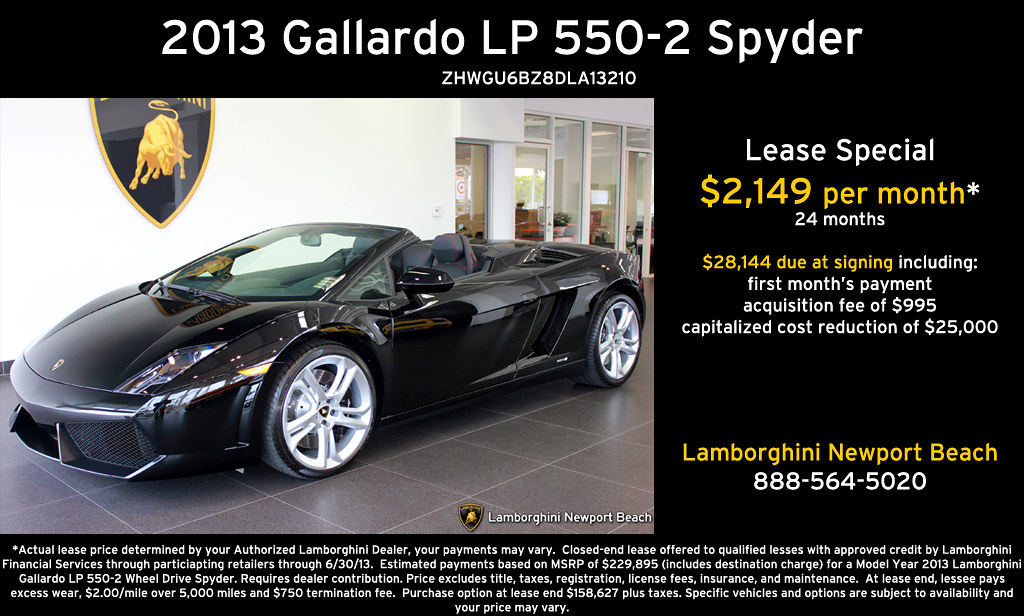This detailed advertisement poster showcases the sleek, black 2013 Gallardo LP 550-2 Spyder convertible. The car, with its top down, features a low-profile design and two doors, exuding an air of luxury and performance. The backdrop is an elegantly tiled car dealership floor with a white wall bearing the Lamborghini logo—a black shield bordered in gold, emblazoned with a striking gold bull. In the upper section of the poster, the model and type of the car are prominently displayed in white text against a black background: "2013 Gallardo LP 550-2 Spyder." Below and to the right of the image, it reads "Lamborghini Newport Beach," while further right, a promotional message indicates a lease special rate of "$21.49 per month." The right side also includes additional leasing information, the amount due at signing, and contact details. The bottom of the poster features fine print legalese, providing all necessary disclaimers and detailed terms of the offer.